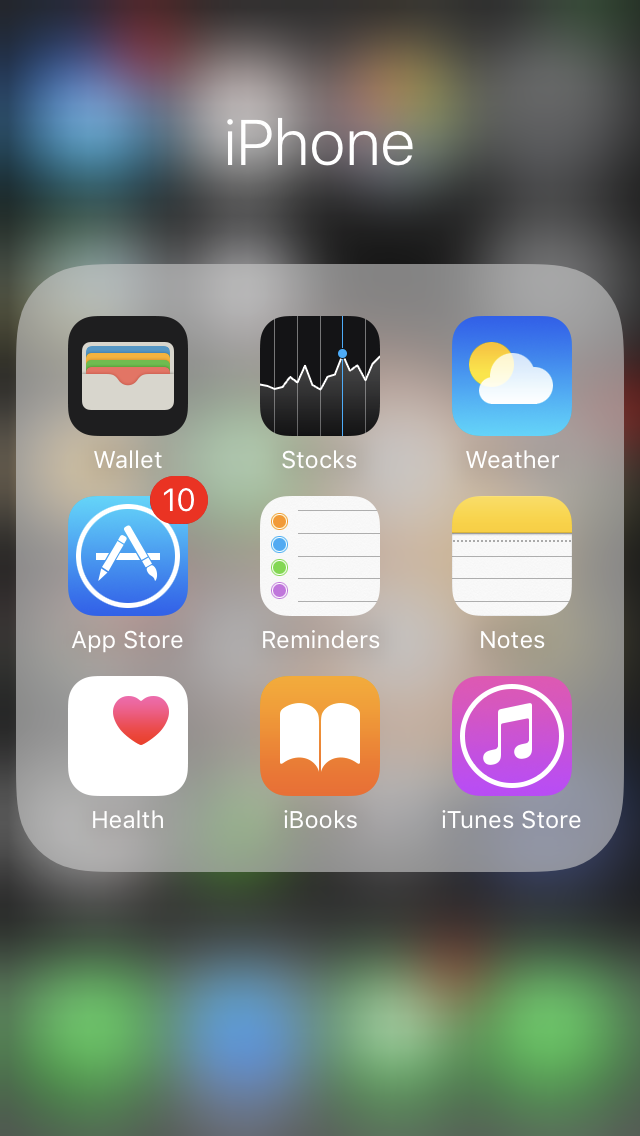The image showcases an iPhone home screen featuring nine distinct apps prominently displayed against a blurred background of obscured app icons. The visible apps include:

1. **Wallet**: Icon characterized by a simulated stack of credit cards in various shades of orange, red, green, and blue.
2. **Stocks**: Includes a white jagged line and a blue line symbolizing stock market graphs.
3. **Weather**: Displays a sun partially obscured by clouds against a blue background.
4. **App Store**: Depicts an 'A' constructed from three pencils or pens, with a small number "10" in the upper corner.
5. **Reminders**: Simplistic icon representing task reminders.
6. **Notes**: Features a yellow-orange header with lined paper beneath.
7. **iTunes Store**: Showcases a large musical note.
8. **iBooks**: Orange icon with the silhouette of an open book represented by two white pages.
9. **Health**: A white icon adorned with a red heart.

The remaining portions of the screen are heavily blurred, rendering the other app icons indistinguishable.